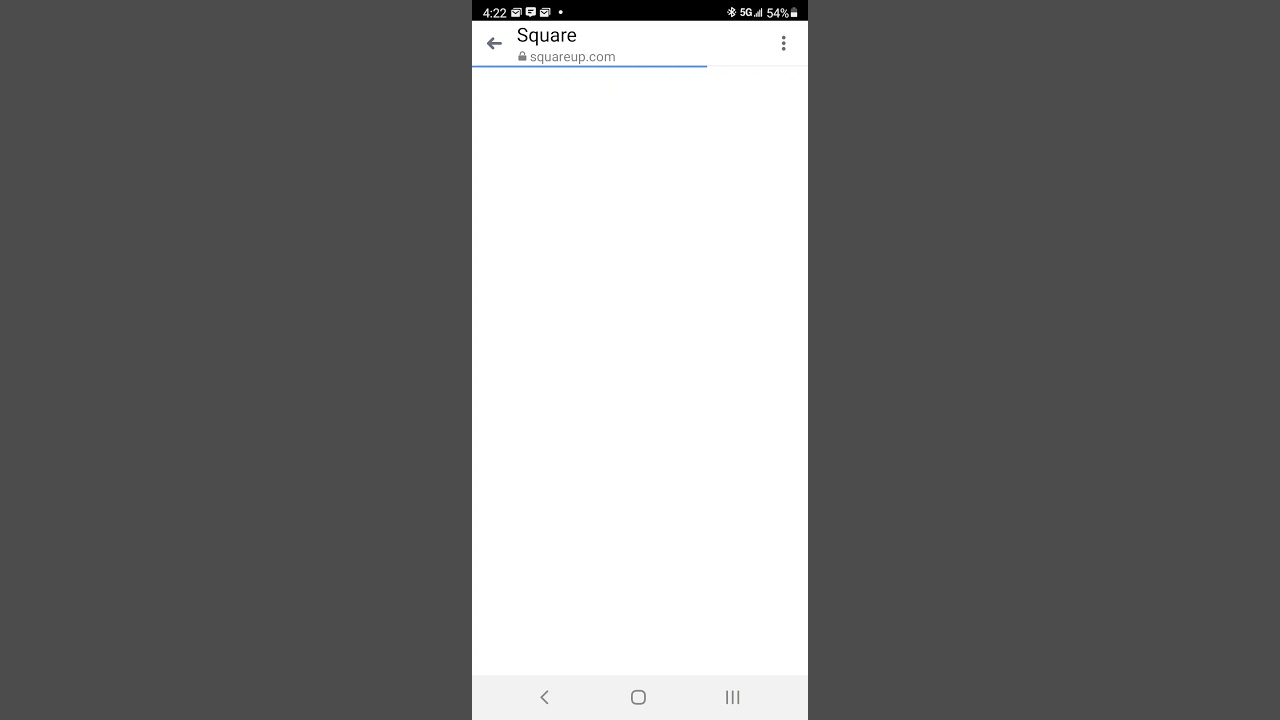The image features a screenshot of a smartphone screen set against a gray background. At the top of the screenshot, a black border displays the time as 4:22, accompanied by three small, unidentifiable icons. On the top right, the status bar shows 5G connectivity with four signal bars and a battery life of 54%.

Below the status bar, the main section of the screen has a white background. Positioned toward the top-left, there is a black arrow pointing to the left next to the word "Square." Directly below that, a lock icon appears alongside the text "squareup.com," indicating a secure connection. A light blue horizontal line is placed beneath this URL information.

To the right of this section, there is a vertical ellipsis consisting of three dots stacked vertically. At the bottom of the screen, a gray strip stretches horizontally across the width. On this strip, a left-facing angle bracket (<) is situated on the left side, a square icon is in the center, and three vertical lines positioned side-by-side are located on the right side of the strip. The remainder of the screen is largely empty, presenting a vast, uncluttered white space.